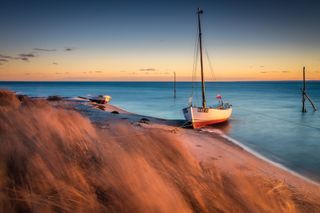The image appears to be an illustrative painting, depicting a serene, rocky, and minimally sandy shoreline. Dominating the foreground on the bottom left is a white sailboat with a red bottom, beached with its sail down. A figure sits aboard, though details are indiscernible. Nearby, another smaller boat rests without a mast or visible crew. The sandy shore may contain some brown or dead grass, indicating a colder season. In the background, the water stretches out in various shades of blue, becoming darker towards the horizon and showing little wave activity. A couple of tall wooden poles jut out from the sea, adding a rustic touch. The sky features a gradient from pale orange to deep blue, suggesting a time around sunset or sunrise, as the sun itself is not visible but the sky remains beautifully lit with a combination of yellow, orange, and bluish-gray tones. This simple coastal scene captures a quiet, almost melancholic beauty.